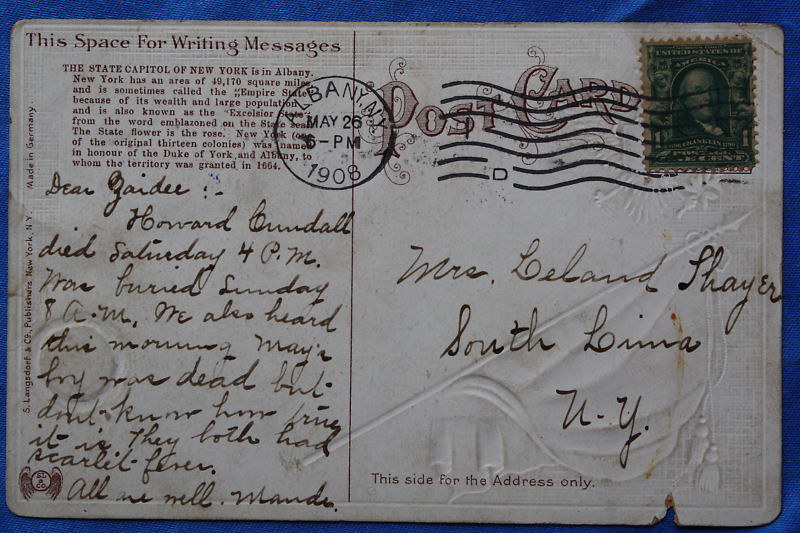This is an image of an old, textured postcard, rich with historical details and tactile features. The back of the postcard bears an embossed texture, likely with ridges that you'd feel upon touching. On the left-hand side, there's a circle with intricate designs, while the right side features a flag on a pole with a pointed end and tassels, partially covered by a green stamp depicting Benjamin Franklin, which is placed in the top right corner.

Prominently printed at the top is the word "Postcard." There is a circular postmark from Albany dated May 26th, 6 p.m., 1908. Below the stamp, handwritten in cursive, is the address: "Mrs. Leland Thayer, South Lima, NY." The printed text on the left side reads, "This space for writing messages." Further printed text includes details about New York State, highlighting Albany as the state capital, New York's area of 49,170 square miles, and its nicknames: the "Empire State" due to its wealth and large population, and "Excelsior" from the state motto.

Additionally, a personal handwritten message in cursive, although somewhat difficult to decipher, begins with "Dear Sadie." It mentions a few somber updates: "Howard bundle died Saturday 4 p.m. Was buried Sunday 8 a.m. We also heard this morning Mays boy was dead, but didn't know him." This detailed and textured postcard offers a snapshot of personal and historical context from over a century ago.